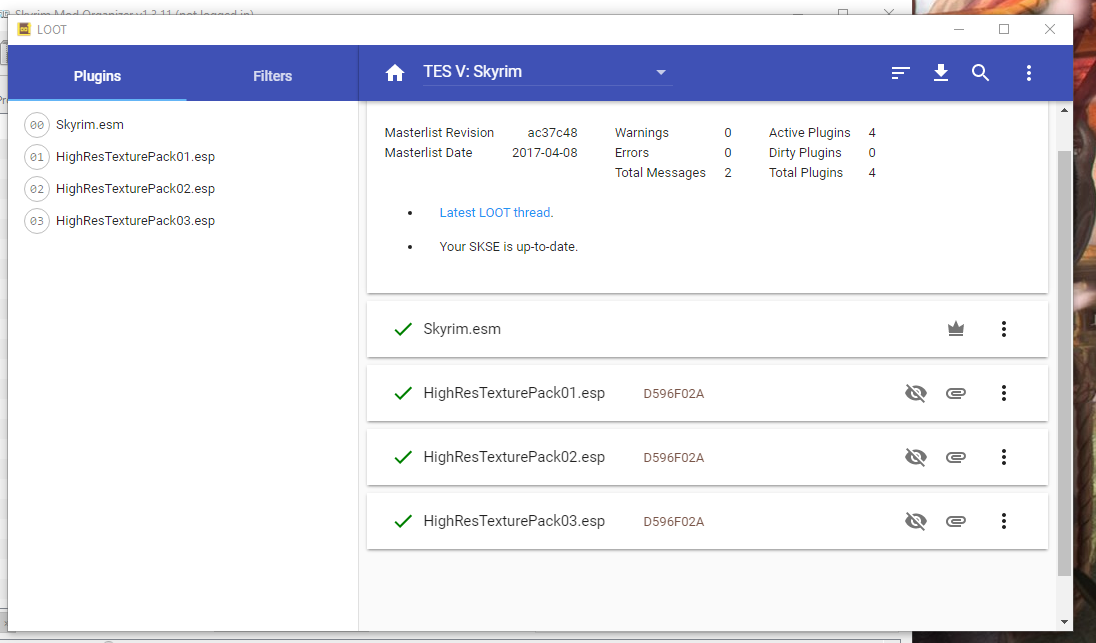The image showcases a pop-up window from the LOOT application on a website. The backdrop of the pop-up reveals fragments of the underlying web page, with visible portions on its right side and the top, including an image of an unknown subject. The LOOT pop-up itself prominently features a distinct logo to the left of the name "LOOT," positioned within a long, horizontal white bar. Below this white bar, a blue strip displays options like "Plugins," "Filters," and a house icon followed by "T as V" and "Sky Skyrim."

Within the pop-up, there are various interactive elements, including icons for search, download, and a three-dot menu symbolizing additional options. The interface also incorporates horizontal menu bars within the white section, where different resolutions and computer terminology are listed. On the left side, these details are arranged vertically, while on the right, they are aligned horizontally.

At the forefront of the display, a blue-highlighted button stands out with the text "Get the latest LOOT," inviting users to click it. The remainder of the information is presented in black text, outlining four categories, each accompanied by green checkmarks for validation. Additionally, there are icons to the right of each listed category.